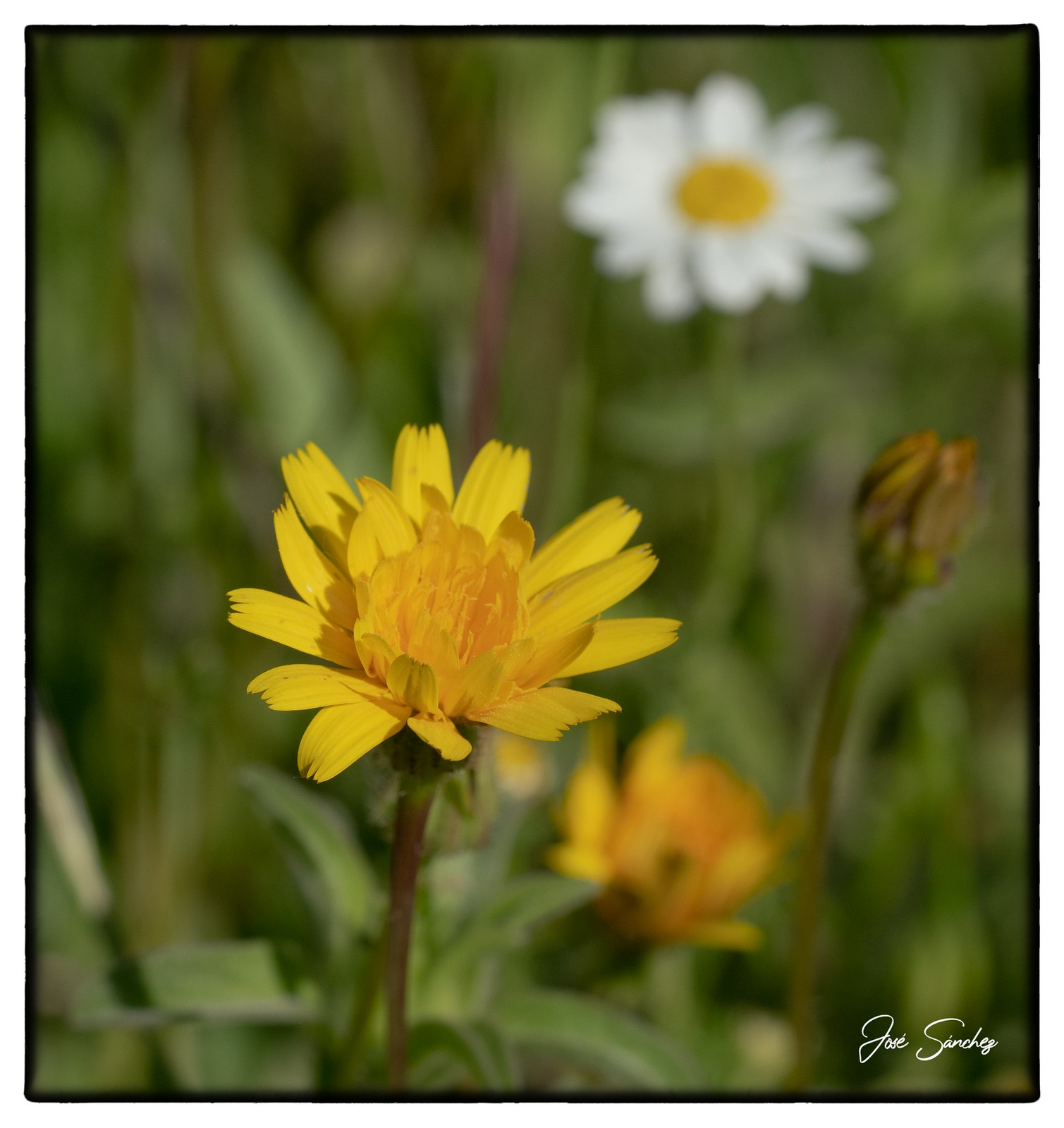The photograph captures a striking yellow dandelion blooming in the center, slightly to the left, its petals starting to unfurl and its center still curled in the budding stage. The image, bordered in black and square in shape, presents a lush background of blurred green grass and additional flora. Notably, in the lower right corner, there is another dandelion that mirrors the one in focus but is out of bloom and partially hidden within the greenery. Above this, a daisy with white petals and a yellow center stands out among the green backdrop, though it too is slightly blurred, indicating it is not the focal point. The scenery is complemented by dark and light greens, along with grays. The bottom right corner contains the artist’s signature in white cursive that appears to read "Jose Sanchez."